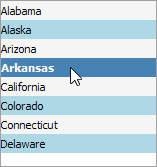The image depicts a dropdown menu listing U.S. states in alphabetical order, starting with Alabama in black text at the top. Following Alabama are Alaska and Arizona, both also in black text. The state of Arkansas is prominently highlighted with a darker blue background, indicating it is currently selected by a white mouse pointer. The selection appears in a manner typical of dropdown menus on websites, possibly for choosing a state for location identification purposes. Continuing down the list in black text are California, Colorado, Connecticut, and Delaware. The backgrounds alternate, with some states on a white background and others on a lighter blue background, emphasizing the standard dropdown menu design.